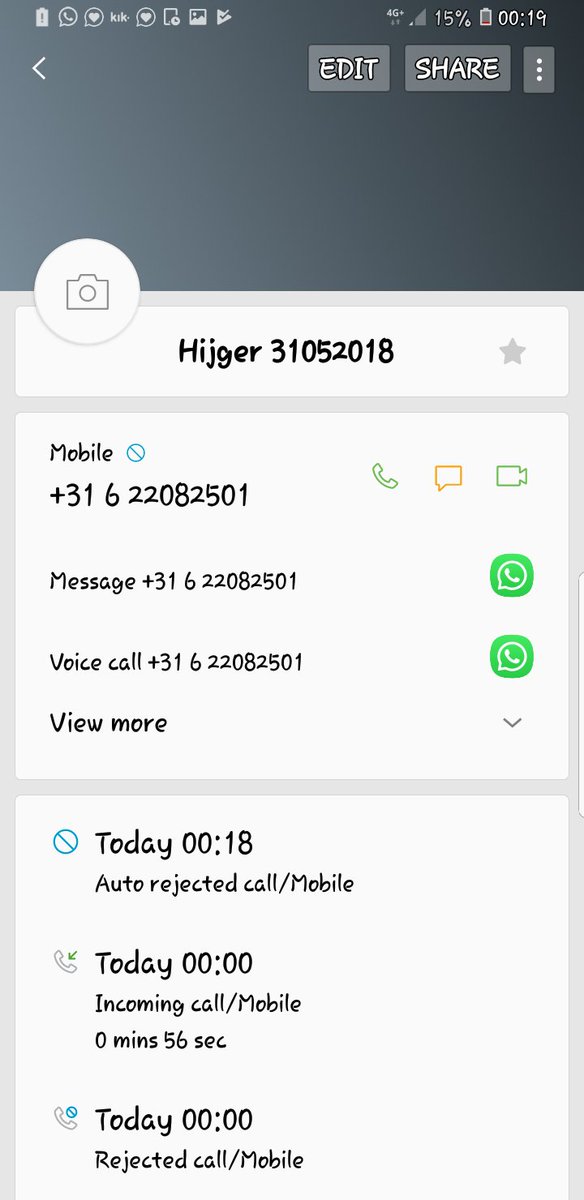In the image provided, the topmost section features a wide gray bar that spans the width of the screen. This bar includes standard phone interface elements, such as battery life, signal strength, and a small white arrow for navigating back to the previous screen. Beneath this bar, at the very center, there are two lighter gray buttons labeled "Edit" and "Share," followed by a small box with a cube shape containing three dots.

Transitioning from the gray bar to a white background, the screen content is divided into three distinct sections. On the left side, there's a circular icon depicting a camera. The middle section, which is narrower, displays the text "HI-JG-ER-310-5201." On the right side, the section showcases a star icon, followed by textual elements reading "Mobile," a phone number "316-220-82501," and options for "Message," "Voice Call," and "View More." 

Below these functional elements, the screen transitions to show the call history for the day, documenting recent interactions associated with the provided mobile number.